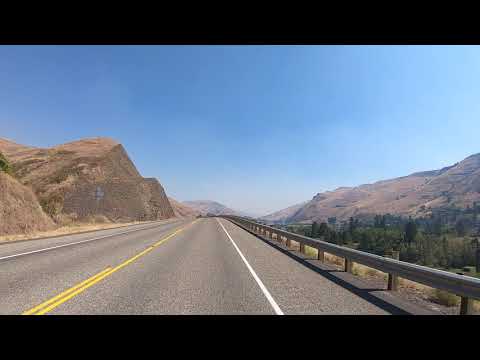This image captures a picturesque roadway scene that seems to be taken from a vehicle, possibly traveling along a highway. The focal point is a two-lane paved asphalt road that stretches forward, marked by solid white lines on both sides and a central divider of yellow lines indicating no-passing and passing zones. On the right side, a short metal guardrail runs adjacent to a narrow shoulder that might be a bike lane, but doesn't offer enough space to pull over completely. Behind the guardrail, a verdant valley filled with evergreen trees extends outward, contrasting with the mostly barren mountainous terrain.

To the left, the road is bordered by large grayish and brownish rocky formations and sandy mountain dunes, adding to the desert-like scape. The mountains on the right appear higher, with their bases covered in greenery and their peaks and distant slopes echoing the orangey hues of the rocks on the left. These slopes partially surround the valley, which is lined with trees that give way to more rugged, tree-less mountains in the distance.

Above, the sky spreads wide and clear, predominantly blue save for a touch of haziness and a few clouds drifting off to the right, evoking a serene atmosphere. The overall scene is one of contrast—between the rocky, barren mountains and the lush valley—against the backdrop of a bright, expansive sky.